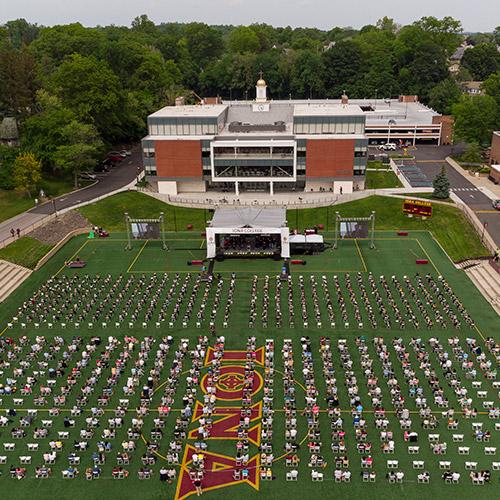The image depicts a spacious and meticulously arranged graduation ceremony taking place on a well-kept football field, most likely during the pandemic. The bright green field features the word "IONA" emblazoned prominently in the middle, and at the front, there is a large stage with two big screens on either side to broadcast the proceedings. Between the stage and the school building in the background, rows of chairs are systematically organized. The back half of the seating is composed of pairs of chairs spaced apart, likely to adhere to social distancing guidelines, suggesting this event is occurring during pandemic times. In contrast, the front rows consist of single chairs spaced farther apart, presumably reserved for the graduates. Families sit behind them, maintaining a respectful distance. The aerial view reveals surrounding greenery and partial bleachers, adding to the sense of a small town academic setting. A tent with officials is visible on the stage, indicating this is indeed a commencement event.